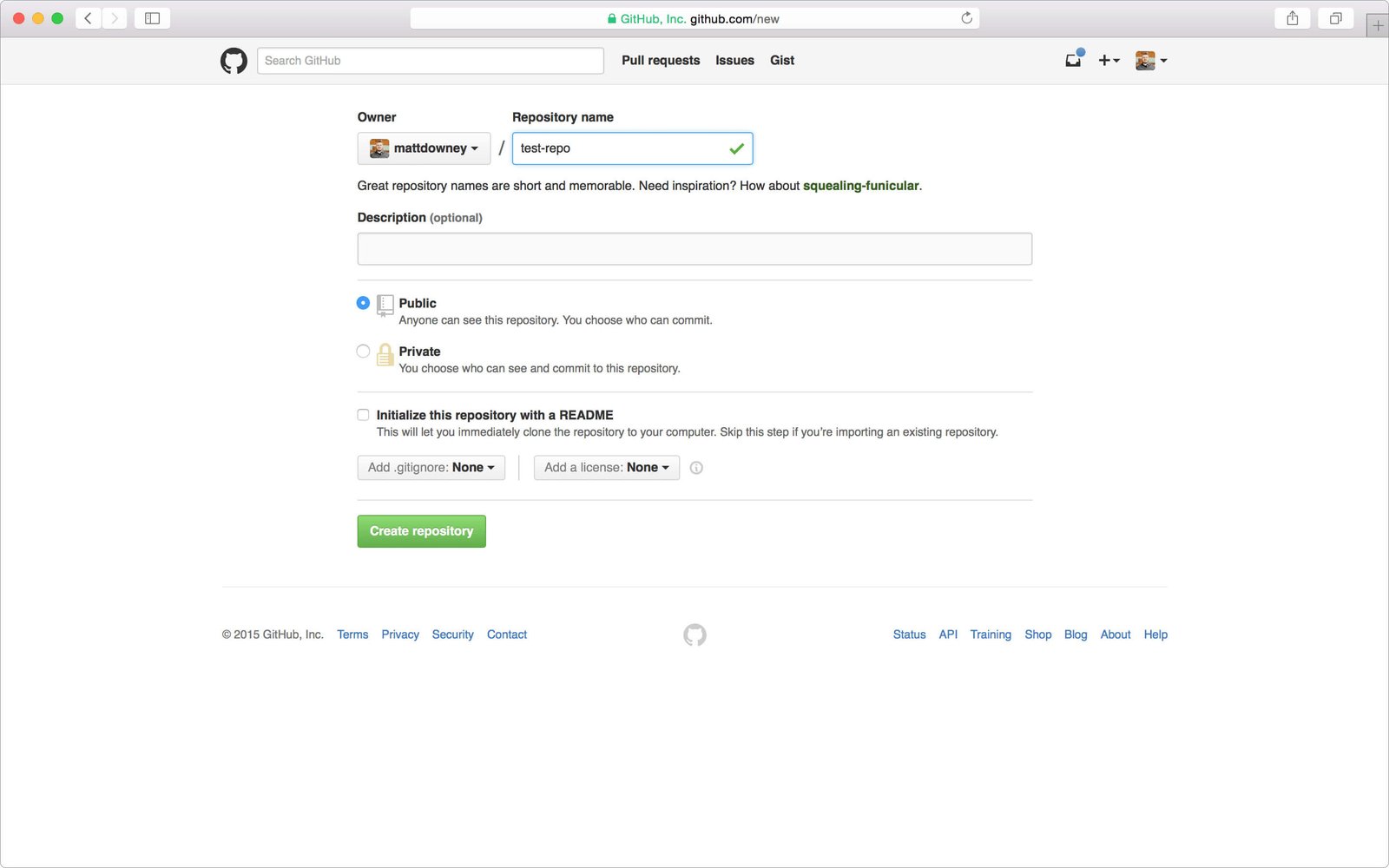A detailed screenshot of a GitHub repository creation page is displayed. The top of the image features a thin gray bar containing icons and navigation buttons: three colored circles (blue, yellow, green) on the far left, navigation arrows beside them, and a central search bar displaying a GitHub URL. To the right of the search bar are buttons for sharing, minimizing, and adding a new tab.

Beneath this bar, the interface shows a white background with the GitHub search box prominently in the middle, accompanied by tabs labeled "Pull requests," "Issues," and "Gists," with additional icons on the far right.

In the center of the page, black text reads "Owner" next to the name "Matt Downey." Adjacent to this, it says "Repository name," where a box outlined in blue displays "test repo," accompanied by a green check mark. Below, a suggestion for repository names humorously proposes "squealing funicular."

Further down, various settings are shown: a description box marked "optional," toggles for "Public" and "Private" (with "Public" selected), and an option to initialize the repository with a README (not selected). Buttons for adding a license and a .gitignore file are also present, both set to "None."

At the bottom, a footer section includes links for "Terms," "Privacy," "Security," "Contact," "Status," "API," "Training," "Shop," "Blog," "About," and "Help," all presented in blue text.